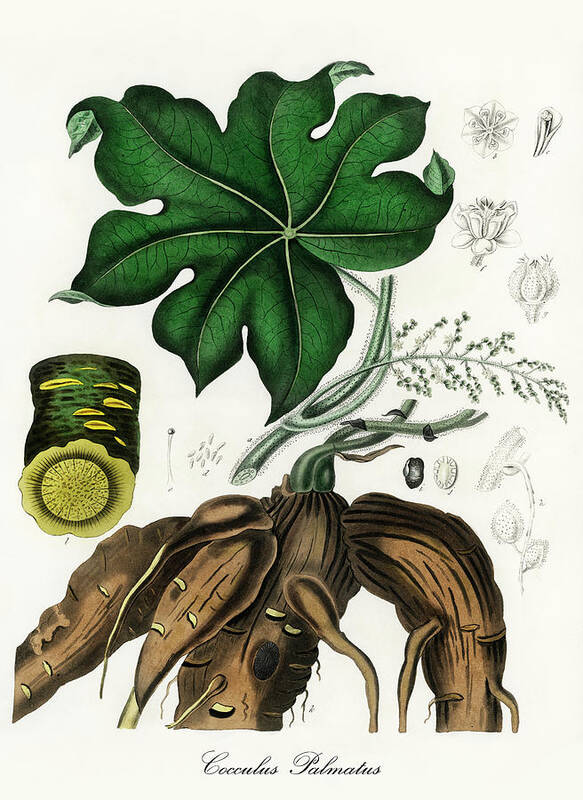The image is a highly detailed drawing of a plant named Coculus palmitus, identified at the bottom of the image. Dominating the top portion are large green leaves with seven distinct petals, characterized by prominent pale green veins. Beneath these leaves on the left side, there is a green, circular tubular structure adorned with red lines. The interior of this tubular part reveals a lighter green color, resembling the shape and look of a kiwi. The bottom section of the image showcases substantial, tuberous roots, with a larger brown root sprouting several smaller ones. Though the plant itself is depicted with fine detail, the root system appears more substantial compared to the above-ground portion. The stem seems slightly furry, and there is an indication that the plant may produce flowers and potentially fruit akin to a cucumber.